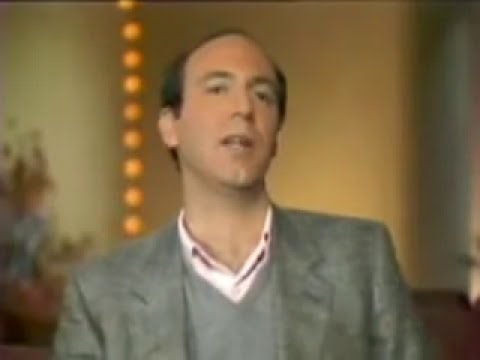This is an old, faded photograph of Gene Siskel, one half of the iconic movie critic duo, Siskel and Ebert. In this image, Siskel, known for his slim build and balding head, is captured wearing a gray blazer over a gray v-neck sweater, which is layered atop a white collared shirt. He is seated in what appears to be a movie theater or cinema-like set, likely part of their famous television show setting, characterized by a beige background with softly glowing neon lights in shades of bright orange and yellow. To his left, there seems to be a plant with red, green, and violet colors adding some life to the scene. Siskel has a mild, almost contemplative expression, with his head slightly tilted and mouth ajar, as though speaking softly. The photograph evokes a sense of nostalgia, capturing the familiar face in a moment of quiet reflection within a backdrop that, though blurred, signifies the world of film critique he was a part of.